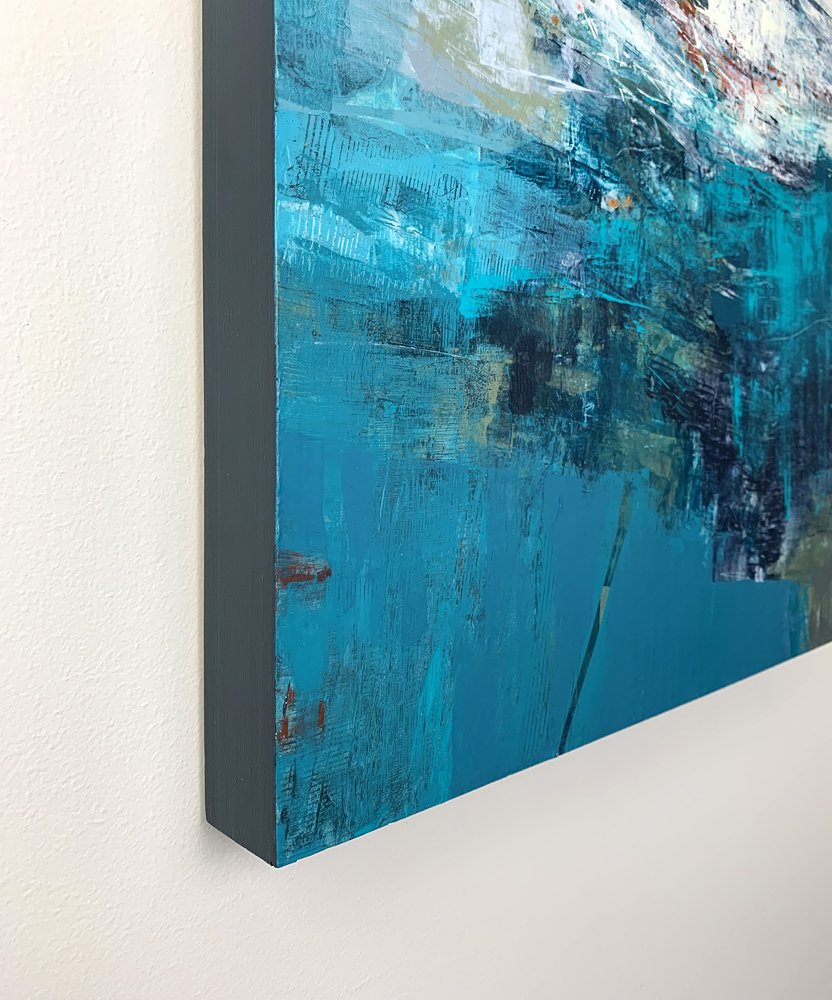This image showcases a thick canvas painting mounted on an eggshell-colored wall, occupying approximately two-thirds of the frame. The artwork is a highly abstract depiction, predominantly featuring various shades of blue, suggesting a dynamic water scene. The canvas is bordered by a dark gray edge and reveals a churning aquatic world replete with swirling whites, deep blacks, and intermittent bursts of teal, sea foam green, and even dashes of orange and red. To the left and bottom left of the painting, splashes of orange evoke an impression of fish amidst the watery depths. The composition suggests movement and chaos, possibly alluding to something recently disturbing the water. A blackish blob with a long stick-like element extending downward adds further intrigue, potentially signifying an undefined creature or object amidst the tempestuous scene.